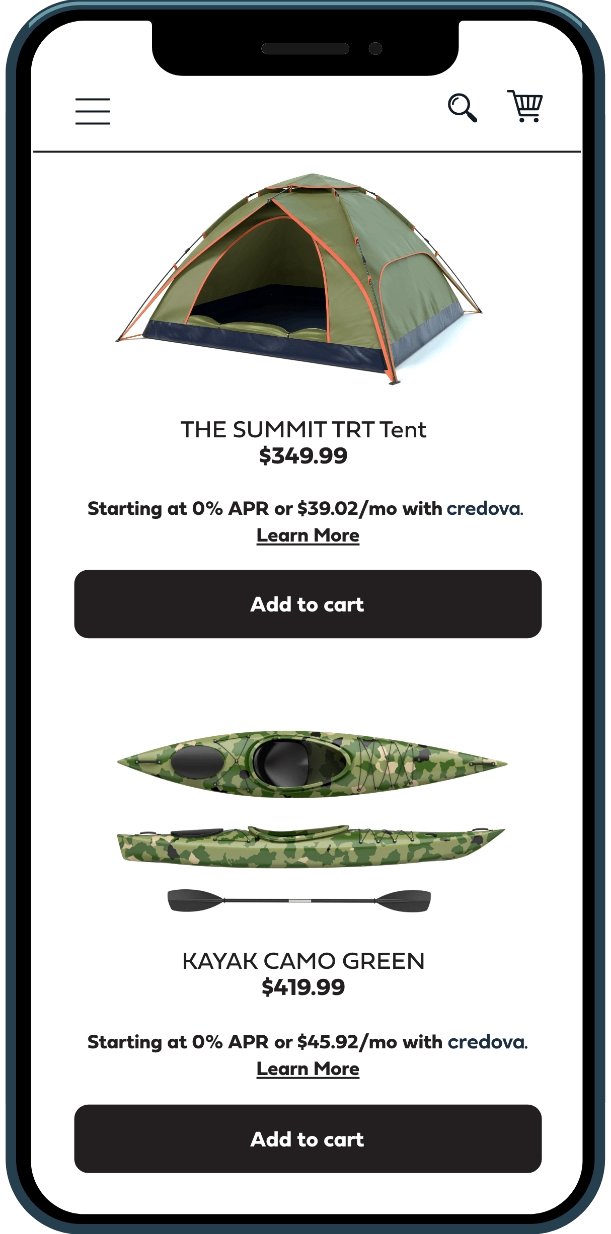A digital image of a sleek, buttonless black-edged cell phone displays a detailed shopping interface. The screen showcases two main products: 

1. **Summit TRT Tent**:
   - **Position**: Center of the screen.
   - **Appearance**: A green tent with visible internal structures including orange holders and a black flooring.
   - **Price and Payment Options**: Priced at $349.99, or available for financing at $39.02 per month with 0% APR through Cordova.
   - **Buttons and Links**: Features two buttons - a large black "Add to Cart" button and a "Learn more" link in small font. The button occupies a significant amount of black space.

2. **Kayak**:
    - **Position**: Below the tent row.
    - **Appearance**: A camo green kayak displayed on its side and face-forward, revealing the interior.
    - **Price and Payment Options**: Priced at $419.99, or available for financing at $45.92 per month with 0% APR through Cordova.
    - **Buttons and Links**: Includes a "Learn more" link, underlined in black to mimic a live link. It also has a large black "Add to Cart" button, similarly occupying considerable space.

The smartphone interface includes additional elements:
- **Upper Left**: Three horizontal lines symbolizing a menu.
- **Upper Right**: Icons for search and a shopping cart.
- **Dividing Element**: A black line separating the top icons from the product listings.

Textual details indicate minor issues with interface design, noting significant areas of wasted space around buttons and links.